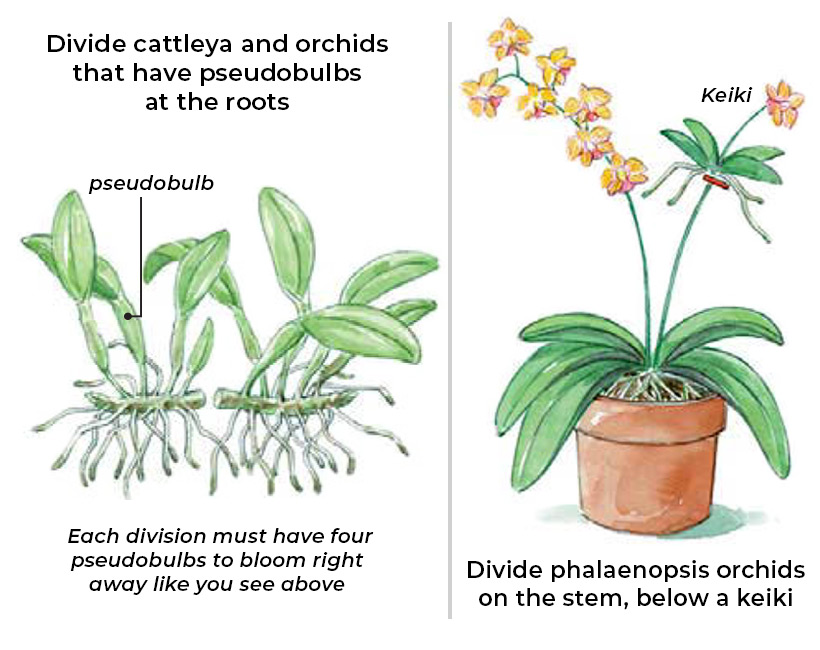The illustration is divided into two sections against a solid white background. On the left is a detailed depiction of two plants attached to a twig or branch, revealing their root systems and green pseudobulbs. Accompanying text instructs: "Divide Catlia and Orchids that have pseudobulbs at the root," with a note at the bottom stating, "Each division must have four pseudobulbs to bloom right away, like you see above." On the right side, a potted plant is illustrated with a brown pot, green leaves, and yellow flowers at the top. The text here labels the top section as "Cakey" and advises, "Divide Phalaenopsis and Orchids on the stem below a cakey," emphasizing proper division techniques for botanical studies. This intricate image, likely from a science book, provides a clear, step-by-step visual guide for dividing orchids, enhanced by descriptive annotations and vivid illustrations.